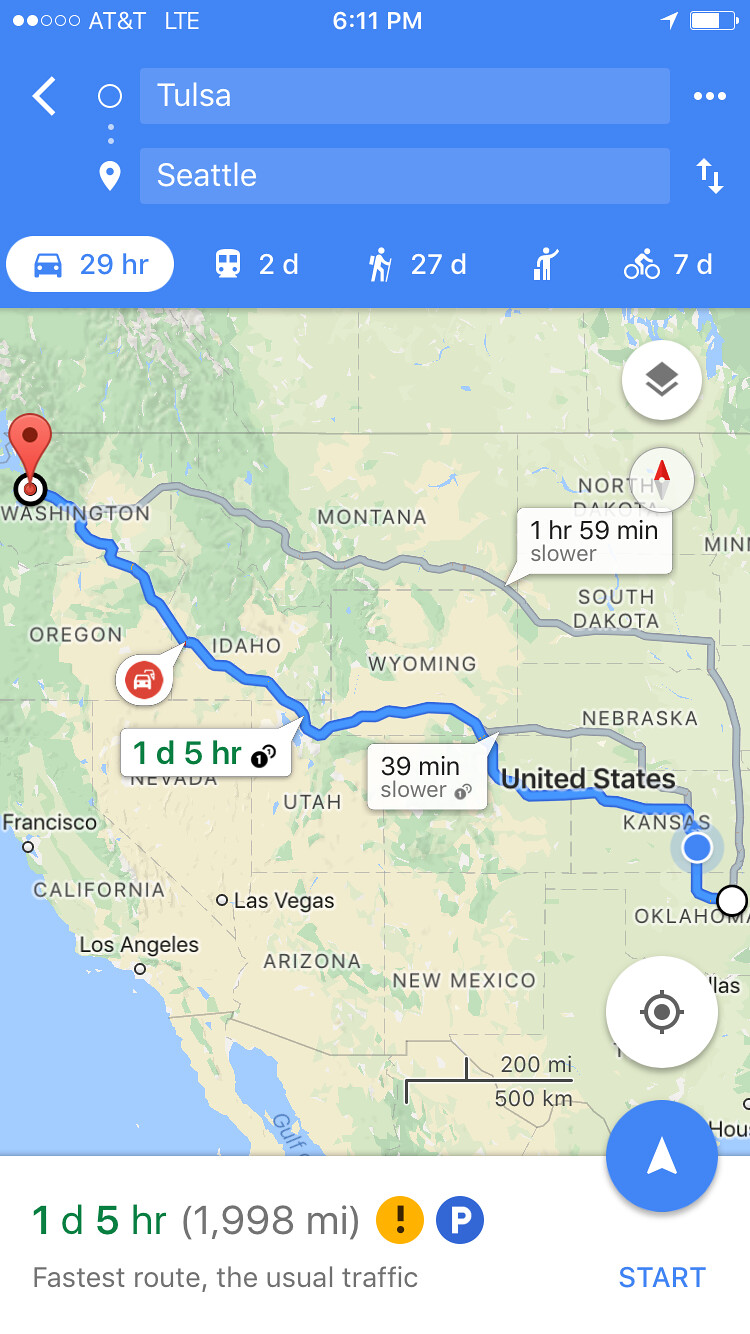This image is a detailed screenshot from a MapQuest-style app depicting the fastest route considering usual traffic conditions. The route spans from Tulsa, Oklahoma to Seattle, Washington, and is highlighted as a thin line stretching westward across the United States. The screenshot has a long rectangular shape with a user interface at the top featuring a bright periwinkle blue background. In the top left corner, it reads "AT&T LTE," while the center of the bar shows the current time, "6:11 p.m." To the right, a battery icon indicates a mostly full charge. The main map details the journey, with labels at the origin, Tulsa, and the destination, Seattle. Below the map, the app provides various travel times: 29 hours by car, 2 days by train, 27 days on foot, and 7 days by bike. At the bottom of the screen, the interface confirms this is the "fastest route" considering "usual traffic," and includes a "start" button for initiating navigation.